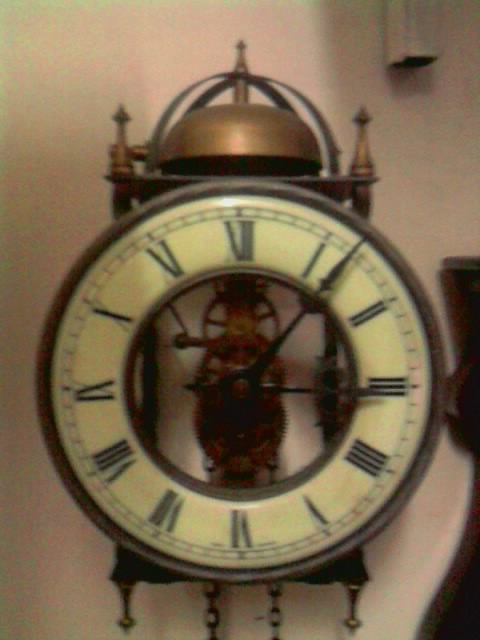This image features an old-fashioned, antique wall clock with a white face and prominent black Roman numerals. The clock shows the time as 3:07, with hash marks indicating the minutes between the 5-minute designations. It has a brass-colored frame surrounding the face, and in the center, there's a hollow section through which the intricate brass workings of the clock are visible. At the top of the clock, a large, dome-shaped brass bell adorned with three upward-pointing spikes and four downward-pointing copper spikes is perched on a platform. Additionally, two chains dangle from the bottom of the clock. The wall behind the clock is a beige color, enhancing the antique aesthetic of the piece.